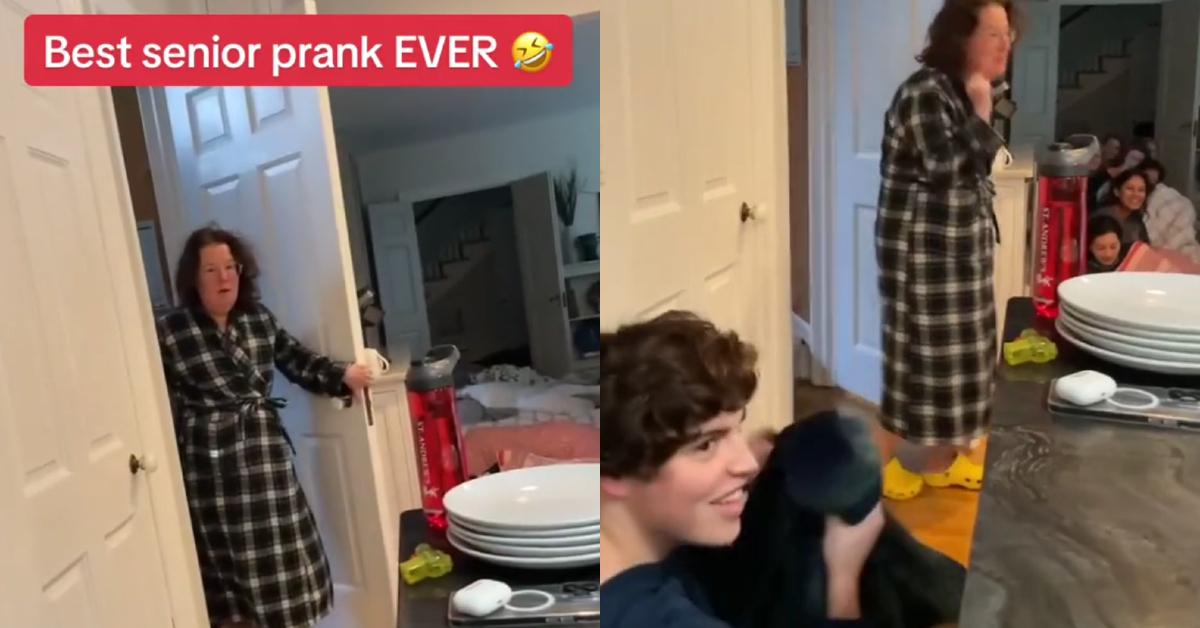The image, likely a thumbnail for a YouTube video or social media post, is divided into two frames. On the left side, a middle-aged woman in a black and white checkered bathrobe and glasses is seen walking through a white door. Above her head, there's a red bubble with white text that reads "BEST SENIOR PRANK EVER" accompanied by a crying laughing emoji. The perspective from behind a kitchen counter reveals part of a messy room with a table, plates, a water bottle, and an open closet. On the right side of the image, the woman appears more surprised as she stands next to a gray-topped kitchen island. Surrounding her are college-aged kids, some crouching and hiding behind the door, others visible with smiling, excited expressions. A young boy with brown shaggy hair is prominently holding a blanket in the foreground, and other children are seen lying in sleeping bags in the background, completing the scene of a well-executed prank.